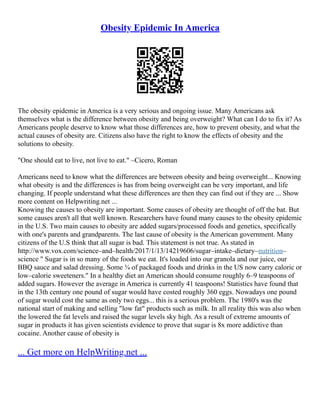The image depicts a densely packed informational page that appears to be low resolution, making the black text difficult to read due to the compression and small size. The page lacks any significant graphic design elements, resulting in a purely text-focused layout on a white background. At the top of the page, there is a black QR code next to an underlined blue hyperlink that reads "Obesity Epidemic in America." Similarly, at the bottom left corner, there is another blue underlined hyperlink that says "Get more on HelenWriting.net." The article focuses on the seriousness of the obesity epidemic in America.